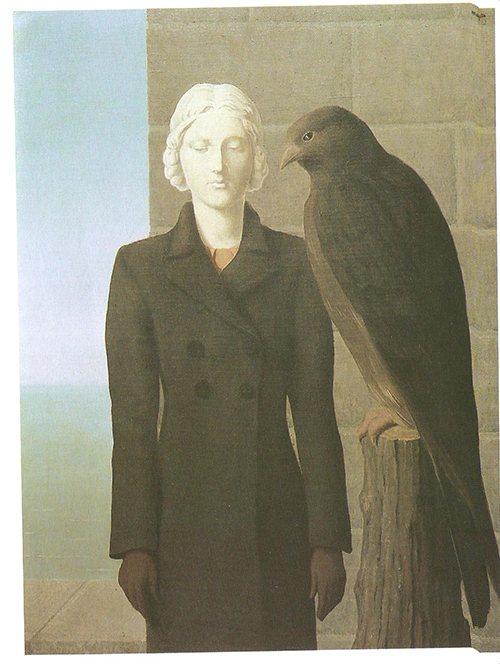This piece of artwork is a vertically aligned, rectangular drawing featuring a female figure with the head of a marble statue, characterized by short, curly hair and downcast eyes. She is adorned in a mid-century modern style, double-breasted black or dark gray peacoat with four buttons on the chest area and gloves on her hands. To her right stands a disproportionately large bird, roughly half her size, perched on a tree stump. The bird is primarily brown with a lighter brown belly, and we see a profile view, including its light brown beak and feet hanging off the stump. In the background, there is a gray stone or cinder block wall that extends from the middle to the upper right, and a blue sky with patches of white occupies the upper left. The overall scene invokes a thoughtful, serene, yet somewhat surreal atmosphere.